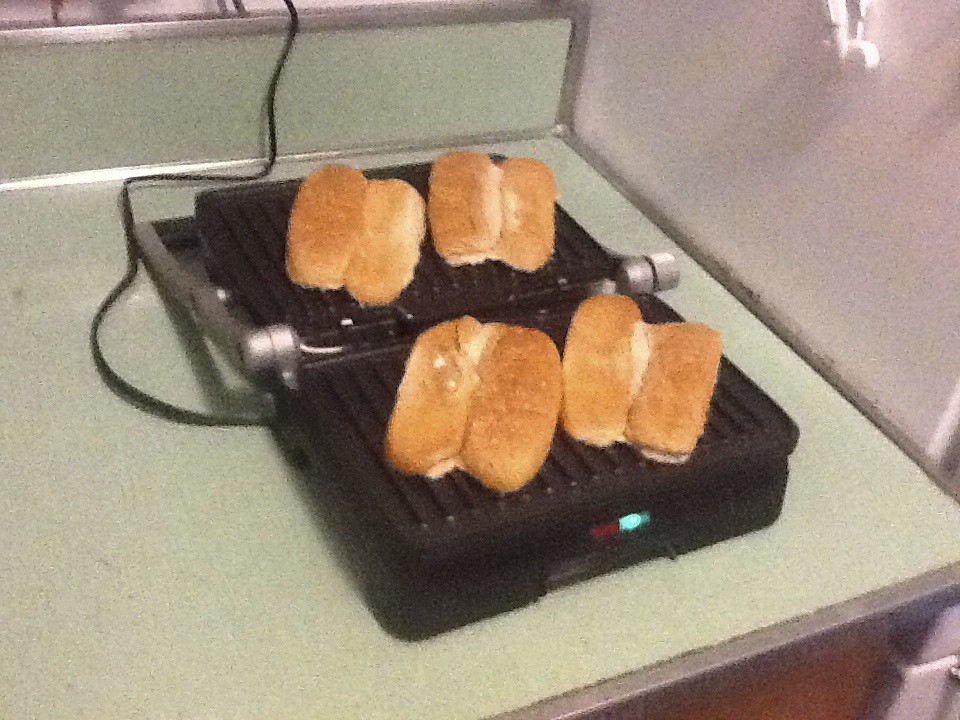This indoor scene features a color photograph, roughly square in shape, capturing a kitchen countertop setup. The light green countertop, possibly Formica, bordered by brushed aluminum, creates a vintage kitchen feel. Positioned in a corner with a grayish silver wall as the backdrop, a black, two-sided grill sits open on the countertop, reminiscent of a panini press or portable burger maker. The grill, equipped with four control buttons and a silver handle pointed towards the countertop's edge, is connected to an unseen power source via a visible plug. On the grill, four hot dog buns are laid out with their white interiors face-down on the grill's surface. The buns are arranged diagonally, with two sets on the top portion and two on the bottom, creating a symmetrical and visually appealing display. The countertop extends to reveal a brown section at the bottom right of the image, adding a contrasting touch to the overall composition.